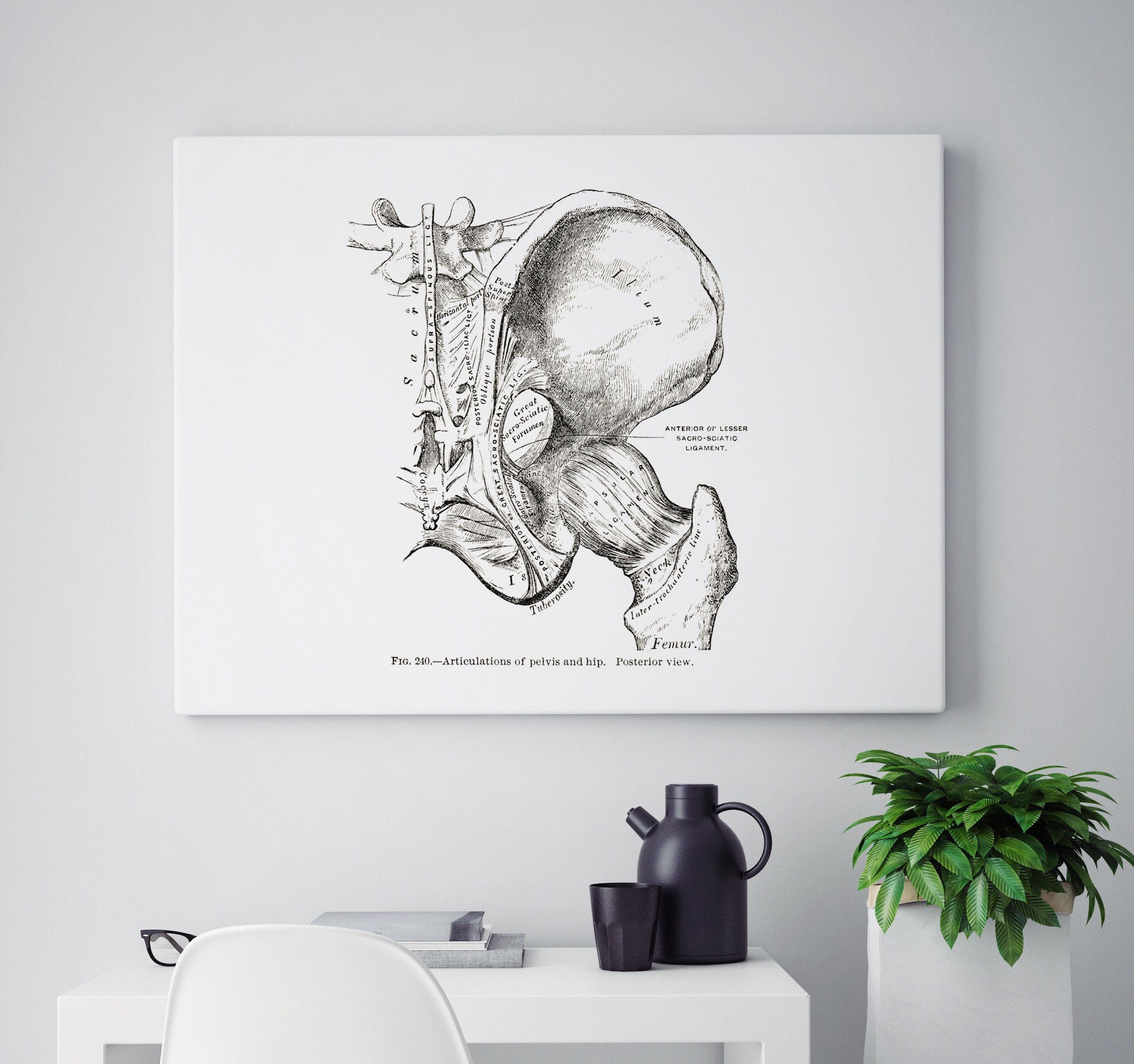The photograph depicts a minimalist office setting with a clean, geometric design. The centerpiece is a white Shaker-style melamine desk, accompanied by a white melamine office chair. On the left side of the desk sits a pair of black-framed glasses. At the center of the desk, there are three neatly stacked books—two gray and one white. On the right, there's a matching black matte tea kettle and cup, emphasizing the monochromatic theme. A white tall rectangular planter holding a vibrant green pathos plant stands to the right of the desk. The backdrop is a white wall adorned with a large, detailed medical illustration of the ilium—the section of the hip bone that connects to the femur, complete with labeled bones. The artwork has a white background with black line drawings and looks like it has been sketched with a charcoal pencil, giving it a precise yet artistic quality. The primary colors in the image are black, white, gray, and green, contributing to its clinical yet aesthetically pleasing atmosphere.